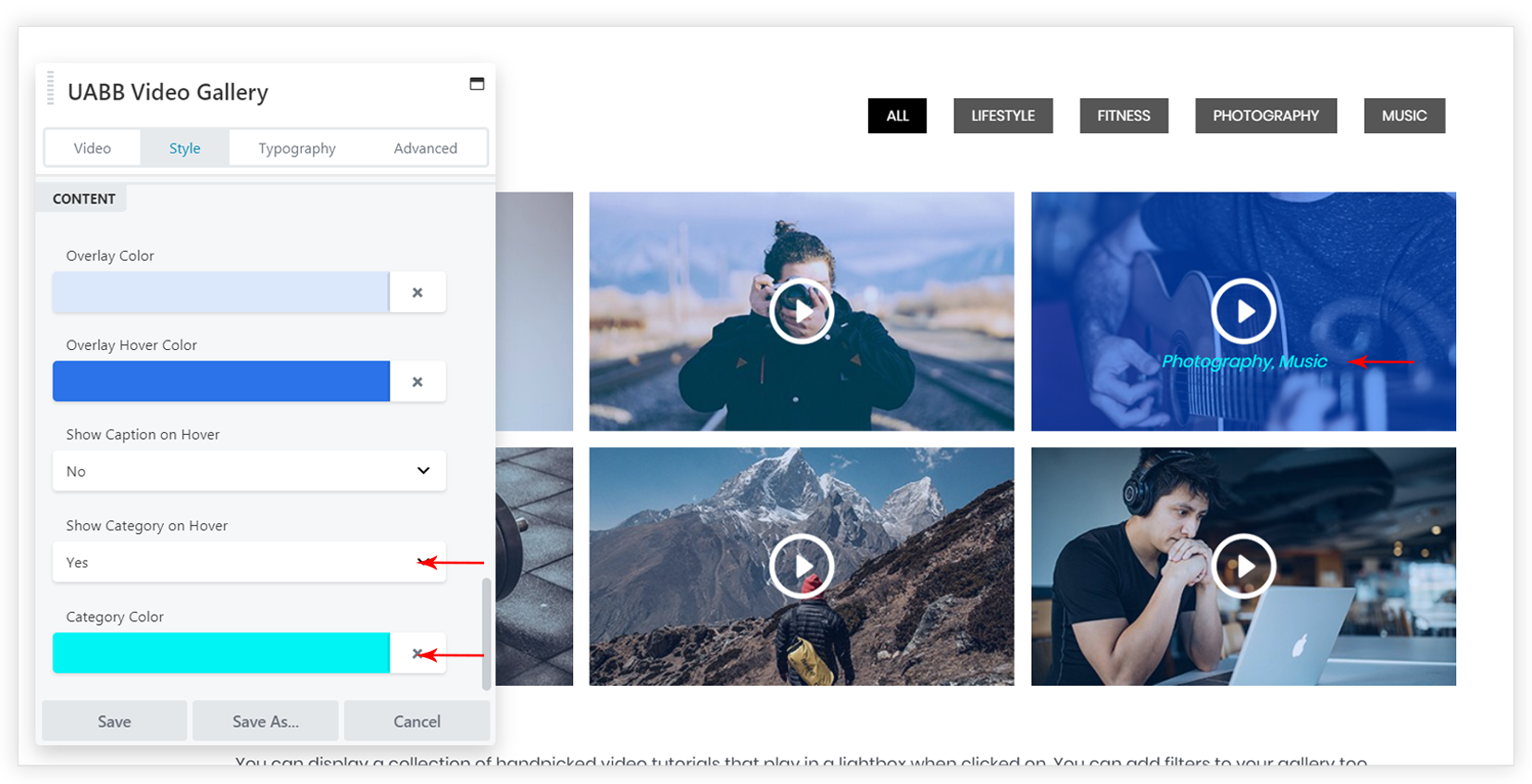This image is a screenshot of a website featuring a UABB Video Gallery module. The website has a clean, white background. Along the left side, there's a tab pop-up panel with a black header that reads "UABB Video Gallery". The panel has several tabs including "Video Style", "Typography", and "Advanced Style". The "Video Style" tab is currently selected.

Within this panel, there are various settings displayed. Under the "Content" section, it lists "Overlay Color" which is set to a light blue and "Overlay Hover Color" set to dark blue. "Show Captions on Hover" is toggled to "No", while "Show Category on Hover" is set to "Yes" – both of these options are highlighted by red arrows. The "Category Color" is defined as a medium-toned blue and is also marked with a red arrow. At the bottom of the panel, there are three buttons labeled "Save", "Save As", and "Cancel".

In the background, partially obscured by the settings panel, are six photographs arranged in a grid. Two photos are mostly covered, but the other four images are visible: one depicts a person standing outside taking a photo; another shows someone playing a guitar with a blue filter overlay; the third image is of a person with their back to the camera standing in front of a mountain range; and the fourth shows a person at a laptop. Each photograph has a white play button superimposed over it, indicating they are video thumbnails.

At the bottom of the image, there is some partially cut-off text that reads: "You can display a collection of handpicked video tutorials that play in something when clicked on. You can add filters to your gallery too."